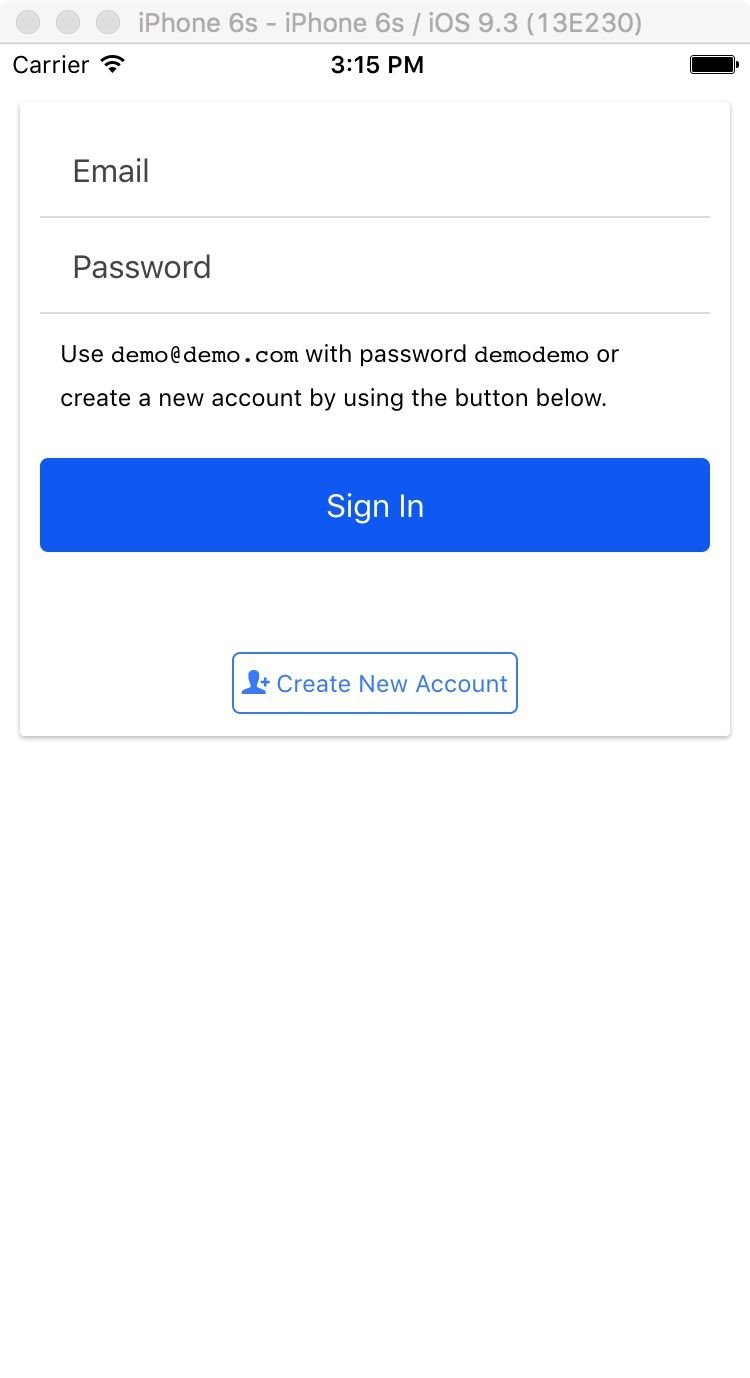A zoomed-in partial screenshot taken on an iPhone displays a view of the upper half of the device's interface. The image includes a light grey triangular section at the top, featuring three uncolored MacBook-style window control buttons for minimize, maximize, and close. Adjacent to these buttons is a grey text label that reads "iPhone 6s - iPhone 6s / iOS 9.3 (13E230)".

Below this section, the typical iPhone status bar is visible, showing "Carrier" in black lettering on the upper left, followed by a Wi-Fi icon, the time "3:15 PM", and a battery indicator.

The main content of the screenshot is a login page, likely a demo version of a website interface. It prompts the user to input an email address above a thin rectangular line and a password below another similar line. The instructions further provide example login credentials, stating "Use demo@demo.com with password demo demo" or offering the option to create a new account by using the button below.

At the bottom of the screenshot, a prominent large blue rectangle button labeled "Sign In" is visible, accompanied by a smaller white-outlined rectangular button below it that reads "Create New Account," featuring a blue icon of a person.